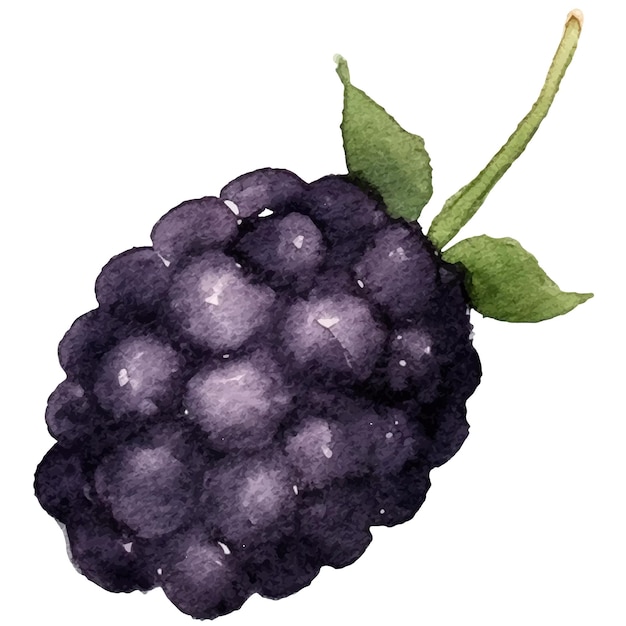This watercolor image depicts a single blackberry, taking up the entire frame against a pristine white background. The blackberry is composed of numerous deep purple, almost black segments, with lighter shades towards the center, giving it a three-dimensional appearance. The intricate detailing makes the berry appear glistening, as if light is reflecting off its surface. Emerging from the top right corner is a green stem, flanked by two rich green leaves, accentuating the berry's natural beauty. The artwork's vibrant colors and meticulous shading make it an ideal piece for a kitchen setting.